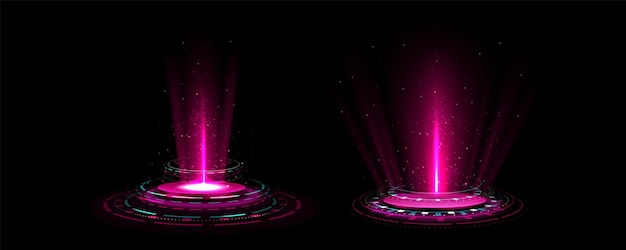Set against a black background, this hyper-realistic digital art features two circular, puck-like lights positioned side by side on the ground, resembling spotlights or possibly futuristic stages. Both lights emit a vibrant array of pink hues, with a bright white stream in the center of each beam. The left light has a more complex design, featuring alternating blue and white dashed outlines and a solid pink core with intermittent white squares. The right light, encircled by multiple green rings and white dots, has a similar but wider configuration with pink hues. Both lights project upwards, with smaller pink lights radiating from the beams, creating an effect that is both otherworldly and visually striking.